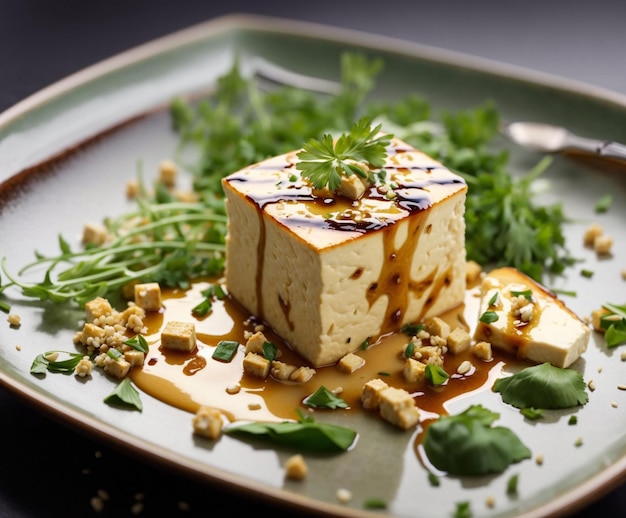The photograph features an artfully presented dish centered around a large, light brown, porous cube that is likely tofu, set on a square, grayish-green plate with a dark rim. A dark brown sauce, perhaps soy sauce with hints of ginger, is drizzled diagonally over the tofu, seeping into the pores and creating darker spots. Atop the tofu rests a small sprig of parsley, and additional parsley and cilantro leaves are scattered elegantly around the plate. Smaller cubes, possibly crumbled tofu or pieces of garlic, adorn the base of the tofu, contributing to the dish's intricate presentation. Behind the central tofu cube, there is a larger gathering of green herbs, adding depth and a touch of freshness to the composition. The entire plate sits on a gray surface, which fades into black, dominating the majority of the background space.